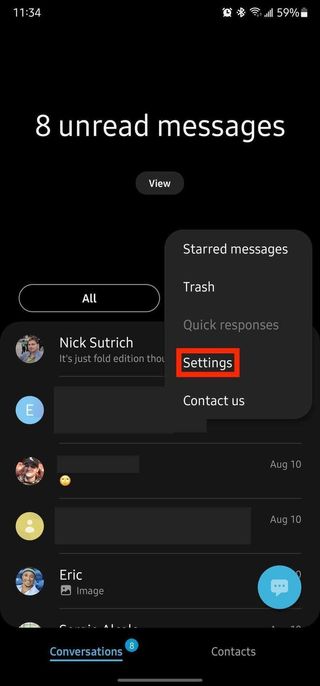The image displays a screenshot of a cell phone interface against a solid black background. The status bar at the top shows the time "11:34" on the upper left, while the upper right displays full Wi-Fi signal bars and a battery level at 59%. Dominating the center is a notification in large white text indicating "8 unread messages," with a small gray box containing the white text "View" directly below it.

Below this, in a gray box, the word "All" is visible. Next to it, there is a circular, blurry photo of a young man who appears to be fair-skinned and wearing a blue shirt. To the right of this photo is the name "Nick Sutridge" followed by the text "It's just fold edition." Beneath Nick's information, there is a light blue letter "E" in a box.

Continuing down, there is another image of a person wearing a baseball cap with the date "August 10th" positioned to the right. Further below, a yellow circle features an icon representing a person, again with "August 10th" to its right. Below is another circle containing an image of a man named Eric. Below Eric's name is what appears to be a black square and a gray square for a photo.

Finally, at the lower left of the screenshot, the word "Conversations" is displayed with a small blue circle containing the number "8."